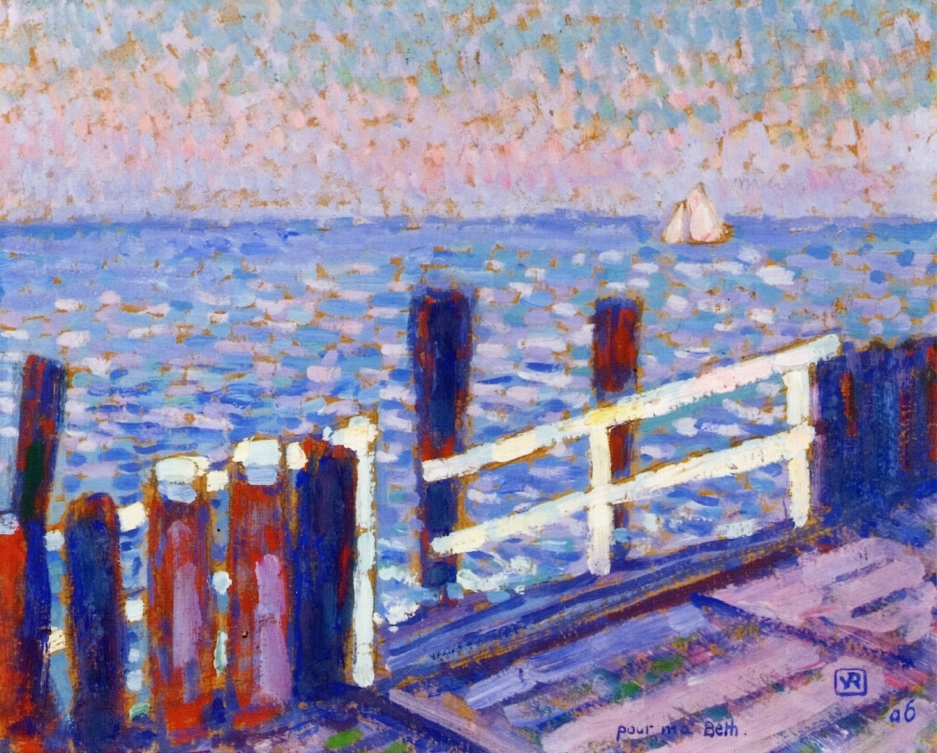This impressionistic painting depicts a serene waterfront scene centered on a wooden dock extending into a body of teal-blue water. The dock is distinguished by circular wooden posts forming the railings, with white lateral boards between them, creating a rustic fence. There are additional posts situated within the water, suggesting an old, weathered structure. The dock features a set of stairs that descend into the water, possibly indicating a boat launch area. The composition includes a white sailboat with a triangular sail in the right background, sailing on the calm waters. The sky above is a light, airy blue, blending softly with the horizon in grayed, muted tones. Bold, visible brush strokes characterize the painting's texture, showcasing the impressionistic style with its emphasis on vibrant, blended colors and lack of sharp lines. In the lower portion of the image, there's a partial inscription that seems to read "P-O-U-R M-A Beth" alongside a logo resembling a connected V and R inside a block, adding an enigmatic touch to this evocative artwork.